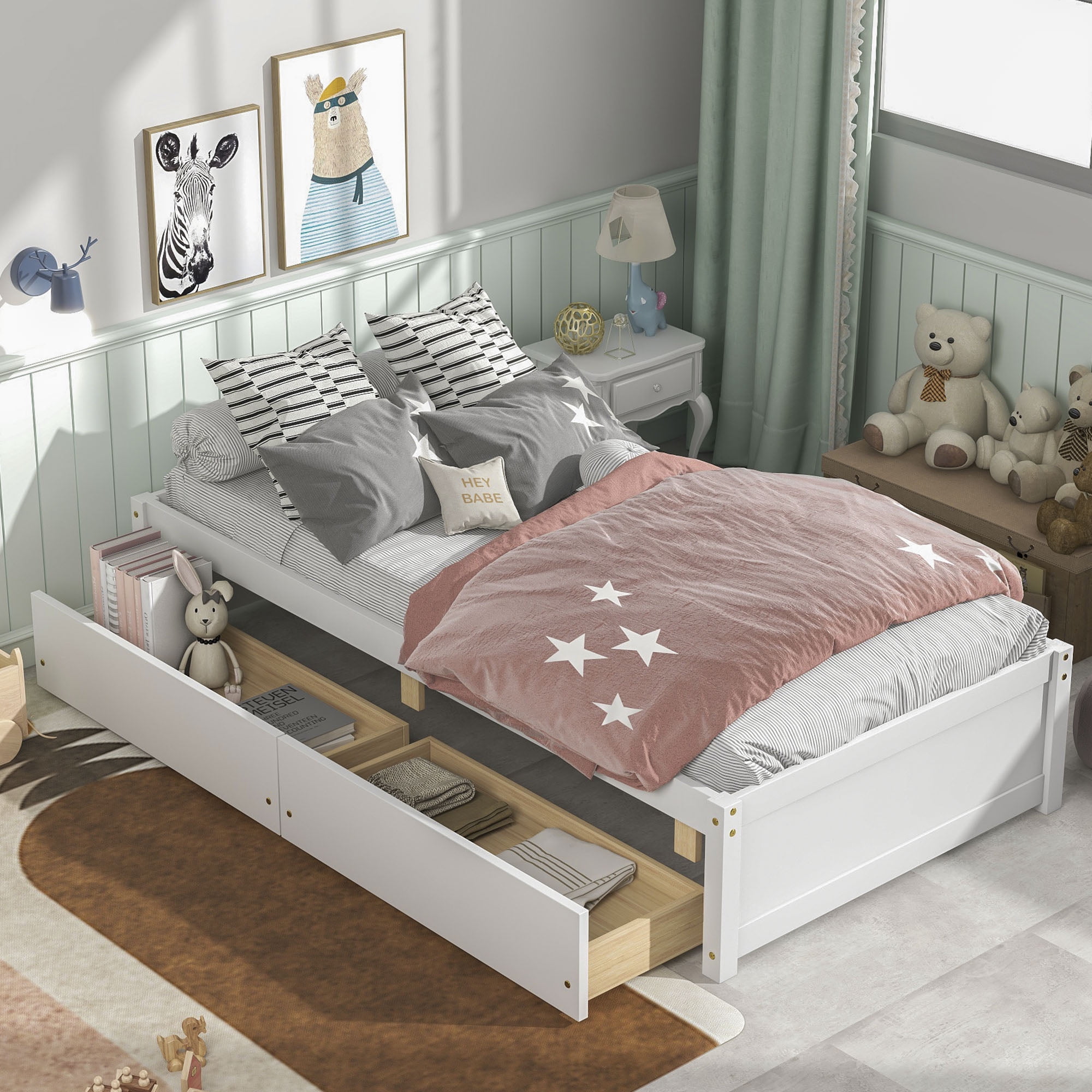This is a detailed photograph of a toddler's bedroom taken from a slightly elevated angle, likely by a tall individual standing beside the bed. The centerpiece of the room is a white bed with a trundle that provides extra storage space, housing books, pillows, and possibly folded blankets. The bed features a charming star theme, adorned with a light pink comforter with white stars, gray pillows with white stars, and additional black and white striped pillows. One small pillow adds a personalized touch with the phrase "Hey, Babe." Adjacent to the bed, a wooden wall mounts a shelf displaying two pictures—one of a donkey and another of a cartoon character, alongside a rabbit statue. Below the window sits a bench holding stuffed animals, including at least three teddy bears. A matching nightstand with a drawer and a blue elephant lamp stands nearby. The room is decorated with green curtains and a brown rug set against a gray floor, creating a cozy and well-organized space for a young child.